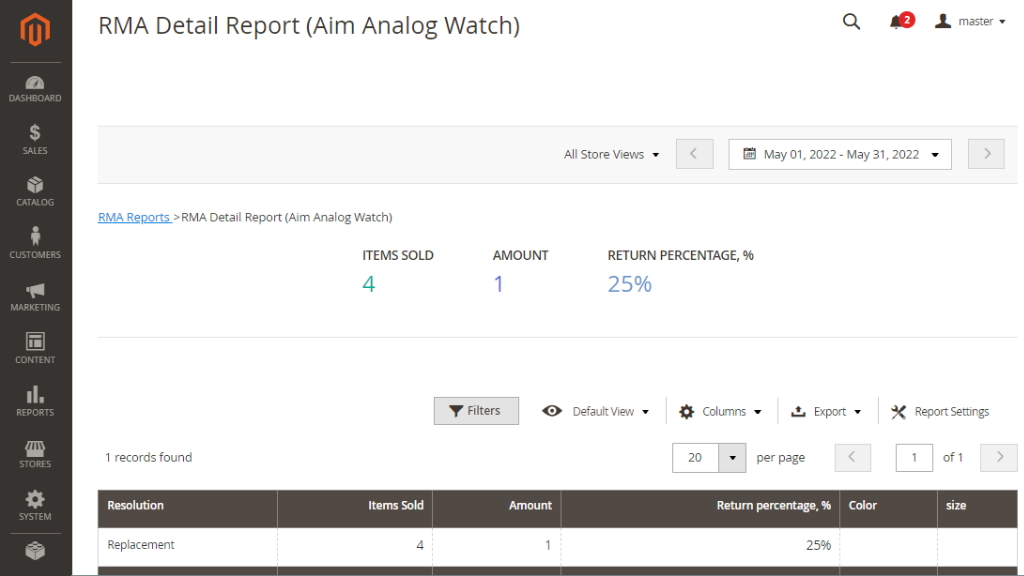This image illustrates the RMA (Return Merchandise Authorization) process for handling returns and defective or malfunctioning products on a website interface. On the left side, a dark gray vertical navigation bar extends from the top to the bottom of the image. This bar is adorned with a red logo box at the top, followed by a series of tabs labeled: Dashboard, Sales, Catalog, Customers, Marketing, Content, Reports, Stores, and System. An additional icon is partially visible, but it is cut off due to the image's cropping.

The central and right portions of the image display a white background. In the upper left corner, the text "RMA Detail Report" is prominently featured, followed by "Aim, Analog, Watch." On the upper right side, there is a search bar accompanied by two notification icons and a user account icon labeled "Master." Below these elements, key performance metrics such as "Item Sold Amount" and "Return Percentages" are provided, offering detailed insights into the RMA process and product returns.